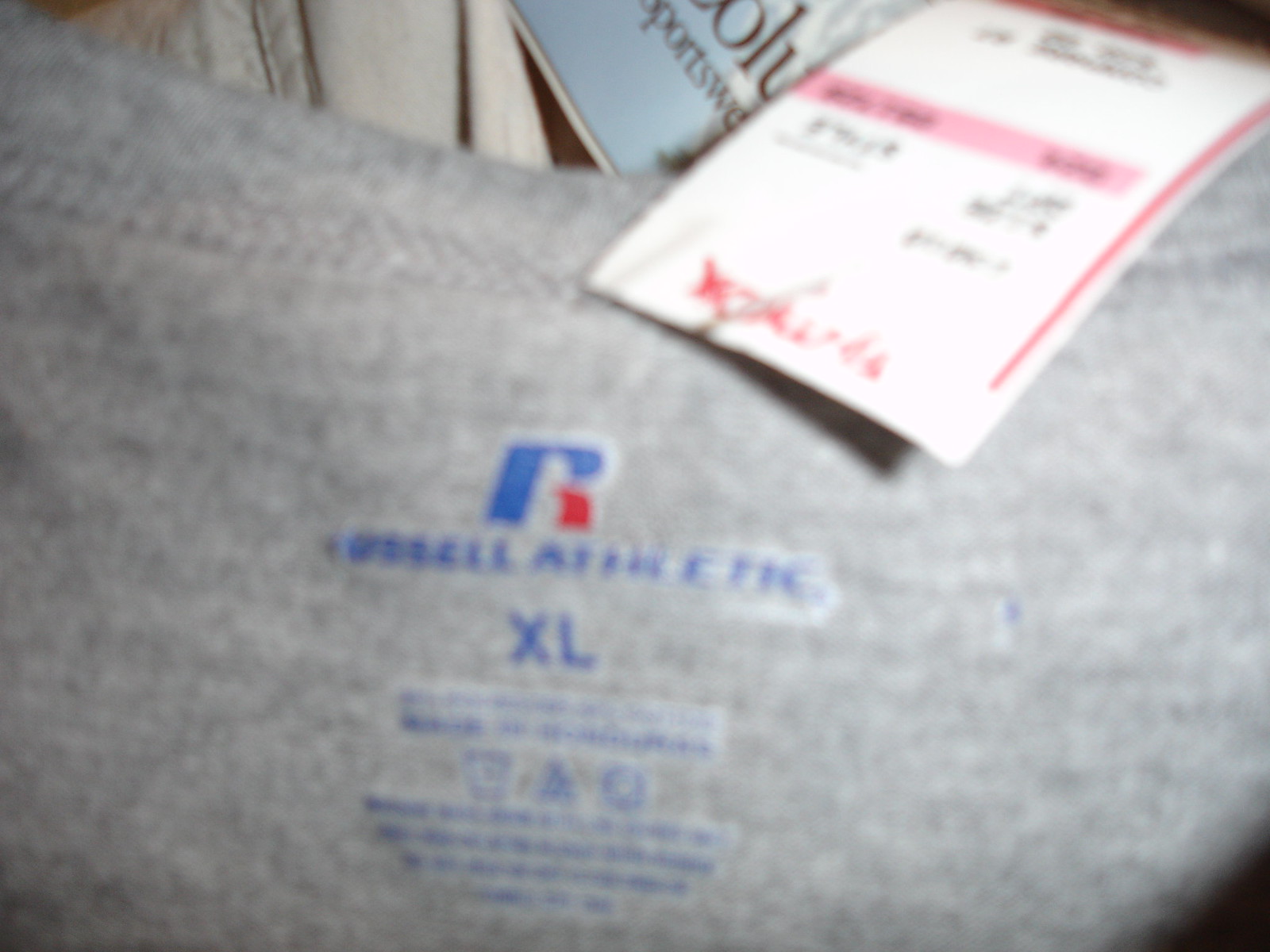This rectangular, landscape-oriented photograph offers a close-up view of the back of a light gray t-shirt with detailed focus on its tags. Dominating most of the frame, the t-shirt features a prominent size tag that showcases a blue and red logo with "XL" printed in blue. In the upper right corner of the image, a secondary tag is visible; it is white with a pink border, adding a touch of contrast to the scene. The background subtly hints at a retail package or box, with the word "sportswear" partially visible, adding context to the t-shirt's environment.